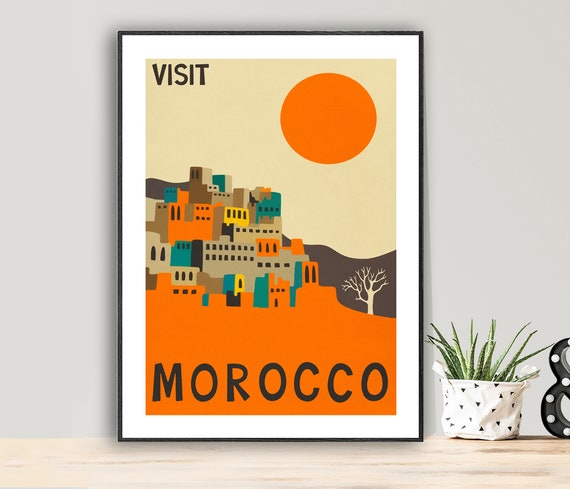A framed picture sits centered on a light wood surface, which has streaks of darker brown and appears to be part of a shelf. The shelf is set against a painted gray wall. The frame is a vertical rectangle with a black border and an inner white matting around the artwork. The picture features an animated depiction of a town on the left side with various buildings in orange, blue, yellow, and gray tones. The background behind these buildings transitions from a tan sky at the top to an orange terrain at the bottom. 

In the upper left corner, the word "VISIT" is printed in black capital letters, while in the upper right, there's a large orange circle symbolizing the sun. Centrally placed towards the bottom, the word "MOROCCO" is prominently displayed in gray, capital letters. To the right of the buildings, on the upper left, there is a gray mountainous area extending towards the middle where a small tree is drawn at the bottom. 

Next to the picture, on the right side of the shelf, sits a white pot with black triangles containing an aloe vera plant with small, thin leaves. Partially off the image on the far right, one can see a fragment of a larger object, possibly a letter or number with lights, suggesting it might be part of a decorative element.